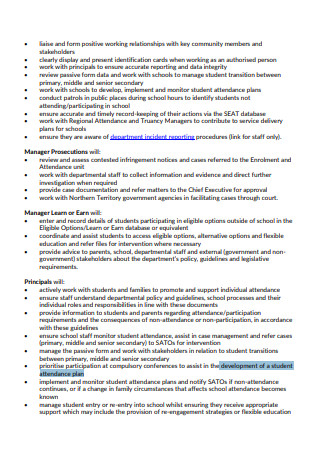The image displays a detailed document forming a lengthy list of information presented in bullet points, categorized under several bold, colored headings. These headings include "Manager Prosecutions," "Manager Learn and Earn," and "Principles," each featuring multiple bullet points outlining various guidelines or instructions. This page appears to belong to a procedural document or terms of service agreement. Notably, a section at the bottom of the page, highlighted in blue, reads "Development of a Student Attendance Plan." The background of the page is white, and all the text is rendered in black.